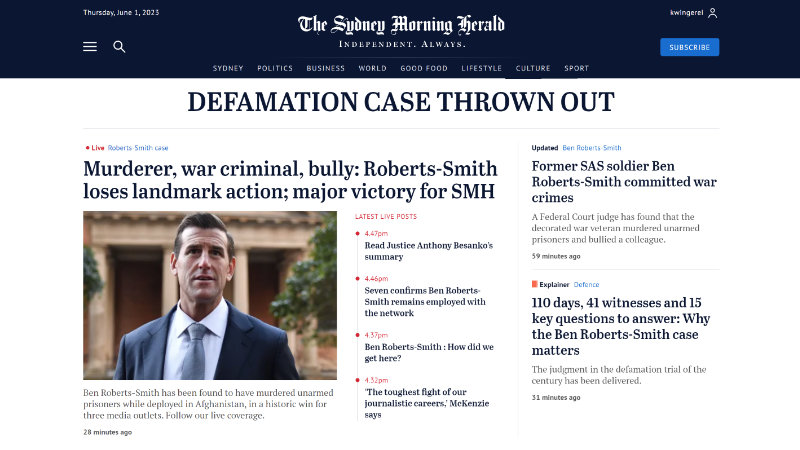In this detailed caption, I describe a news article page from The Sydney Morning Herald, predominantly featuring information about the defamation case involving Ben Roberts-Smith:

---

The top portion of the webpage features a dark background, which seems to be either navy blue or black. In the upper left-hand corner, there is white text displaying the date: "Thursday, June 1st, 2023." Adjacent to it, there appears to be some text that reads "K-Wing-E-R-E-L," possibly indicating the signer.

Below this, the next row contains three white lines and a white magnifying glass icon for search purposes. Centrally positioned on the page, there is the publication's logo, reading "The Sydney Morning Herald, Independent. Always." in white text. Next to it, in a blue and white box, is a subscription button labeled "Subscribe."

The navigation bar below features clickable tabs in white text for different sections: Sydney, Politics, Business, World, Good Food, Lifestyle, Culture, and Sport.

The background then transitions to white, prominently displaying the headline in bold, black capital letters: "DEFAMATION CASE." Following this is a thin gray line separating the headline from the subheader beneath, which reads: "Murder of a War Criminal: Roberts-Smith Loses Landmark Action, Major Victory for SMH."

Beneath the subheader is a photograph of a man wearing a white shirt and blue tie, captioned: "Ben Roberts-Smith has been found to have murdered a prisoner while deployed in Afghanistan and has started going for three media outlets following live coverage." This line of text indicates that the information was updated 28 minutes ago.

Additionally, the accompanying text highlights: "Former SAS soldier Ben Roberts-Smith committed war crimes," including detailed statistics: "110 days, 41 witnesses, and 15 key questions to answer—Why the Ben Roberts-Smith case matters."

---

This descriptive caption accurately compiles and organizes all key information presented in the narrative.